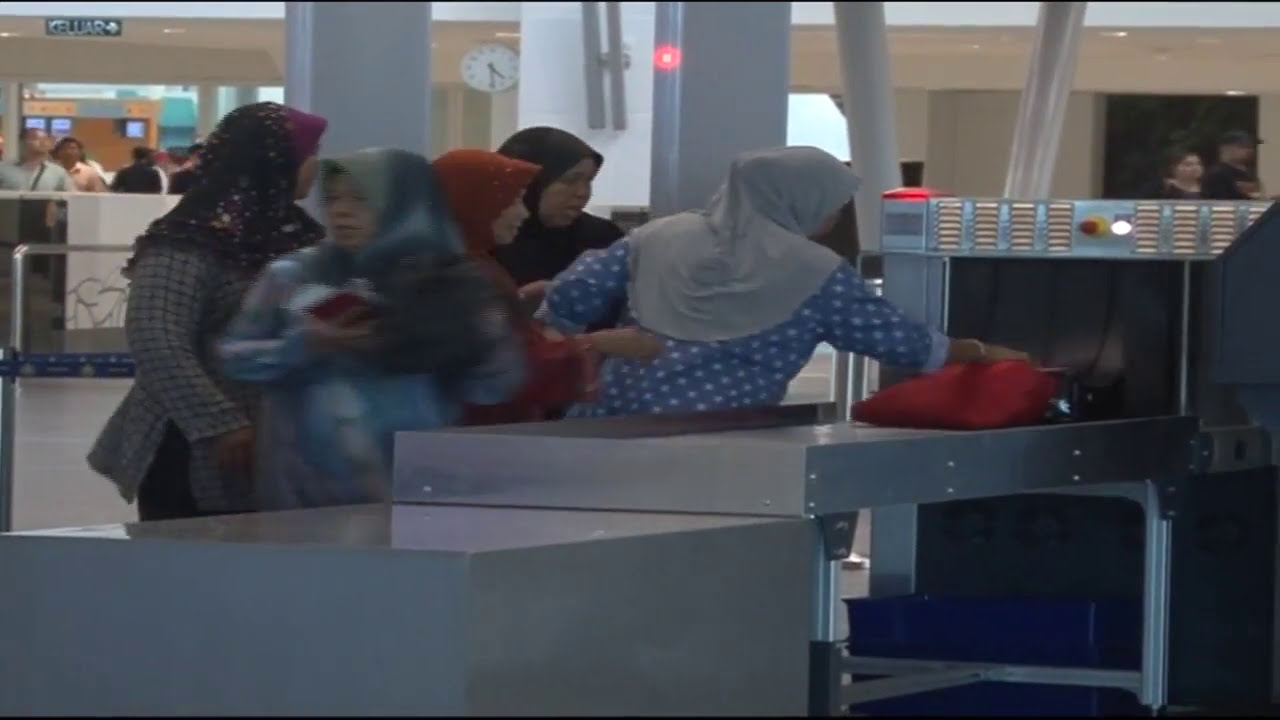The image depicts an airport terminal bustling with activity. The focus is on five women, who appear to be of Middle Eastern descent, dressed in traditional attire with head coverings. Closest to the baggage scanner, a woman with a white head covering and a blue polka-dot long-sleeved tunic is either placing or retrieving a red bag from the x-ray machine. Beside her, another woman wears a black head covering, while the third dons a red head covering. The fourth woman, with a black and purple head covering, is dressed in a dark gray, striped tunic. The fifth woman, slightly blurred due to movement, wears blue and gray head coverings and seems to be turning away. The background shows multiple people walking in the terminal, a hanging clock, large windows, railing, and supporting pillars indicating a spacious environment. A female and a male figure, with the male wearing a hat, stand in the distance, adding to the hustle and bustle typical of an airport setting.